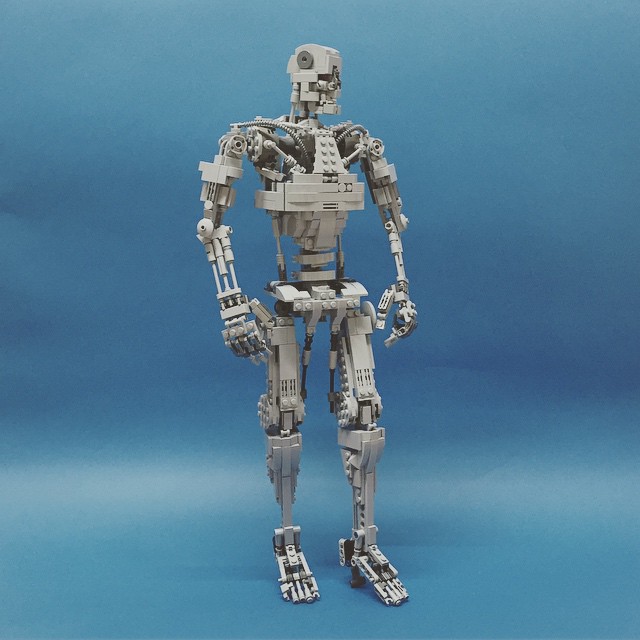This is a studio shot featuring a detailed mechanical robot that resembles a skeletal figure. Set against a blue background with varying shades and hints of white, the robot has a human-like form with distinct features including two legs, arms, a skull-like head, and a torso. Constructed primarily from gray pieces that appear to be Lego blocks, the robot evokes a likeness to the iconic Terminator. The robot stands upright, facing and looking towards the right, with visible mechanical components intricately forming its body, arms, and legs. Notably, it has a network of large wires connecting the chest to the shoulders, articulated joints at the knees, hips, and elbows, and detailed hands and feet with individual fingers and toes.